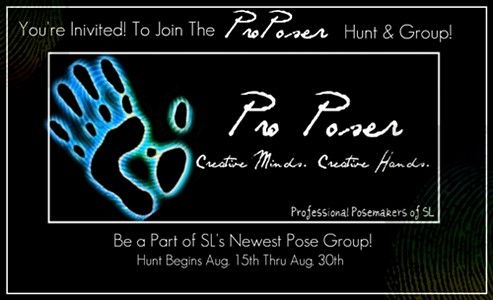This invitation features a sleek black background in landscape orientation bordered by a thin white stripe. At the top, white cursive text reads, "You're invited to join the Pro-Poser Hunt and Group." Beneath this, on the left side, there is a handprint encircled by blue lines, adding a distinctive design element. Adjacent to the handprint, in the same white cursive font, it says, "Pro-Poser." Below this, another set of cursive text proclaims, "Creative Minds, Creative Hands," followed by, "Professional Posemakers of SL." At the very bottom, in clear text, the invitation details, "Be a part of SL's newest pose group. Hunt begins August 15th through August 30th."